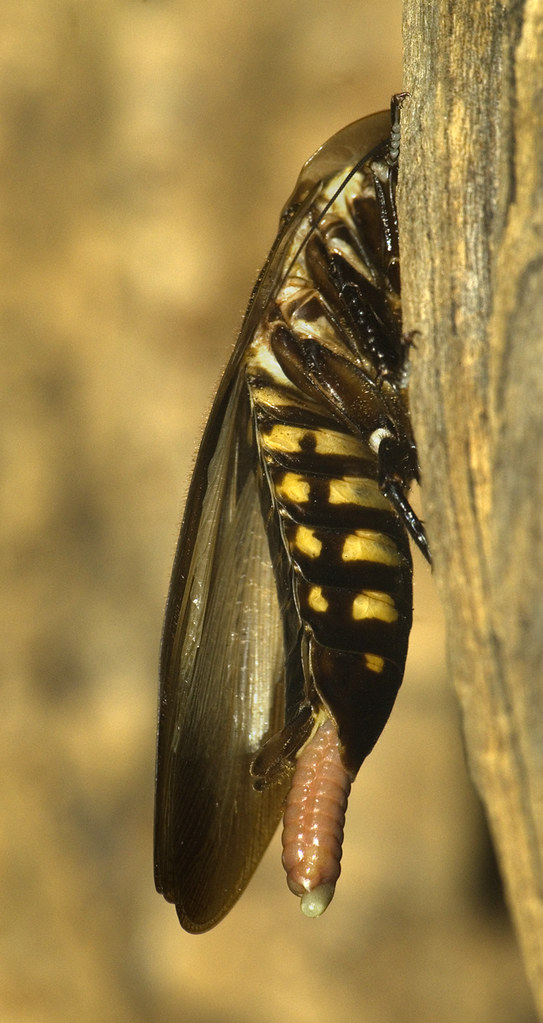This vertically aligned rectangular image captures a nature scene featuring an insect in a wooded area. The background is predominantly composed of out-of-focus, brown-toned leaves and trees, contributing to the natural, outdoor setting. Dominating the right side from top to bottom is a gray and tan piece of wood, likely the bark of a tree, providing a detailed texture in the foreground.

Attached to the middle of this branch-like wood is a large insect, evocatively displayed in close-up detail. The creature resembles a locust with its hard shell near the head, elongated translucent wings extending from its back, and dark black legs gripping the tree. Its torso or thorax exhibits distinct yellow and black stripes, segmented into rounded sections that grow smaller towards the rear. 

Uniquely, emerging from the bottom of the insect is a peculiar, light tan, worm-like entity adorned with green highlights and ending in a beige tip. This feature suggests the insect is undergoing a form of metamorphosis. The overall effect is a striking, vivid depiction of the intricate and often unseen processes of nature.